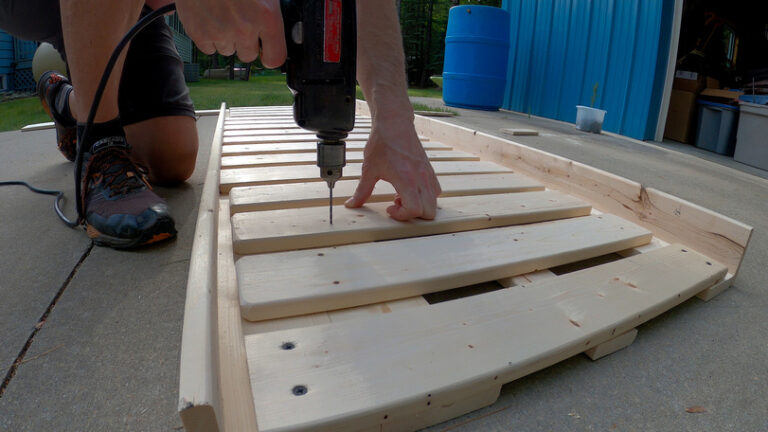In this ground-level photograph, we see a detailed scene of a man working with a drill on a wooden structure. The image is taken from across a concrete walkway that starts at the bottom left corner, rises diagonally upward, and then descends midway through the frame before continuing off to the right. Adjacent to the walkway on the left side, lush green grass extends halfway across the image, lending a touch of nature to the industrial setting.

A blue building partially appears on the left side, contrasted by the man's legs prominently positioned in the upper left quadrant. His right leg is bent, with his shin angled downward and his foot flat on the ground, facing the camera. He is wearing black shoes and black socks. His left knee is on the ground, with the foot directed backward and to the left. He is dressed in black shorts, and his upper body is slightly bent over his work.

The man is holding a black drill with his right hand, directed downward towards a wooden rack. His left hand stabilizes the wood as he drills. The wooden structure features slats running from the bottom right corner upward and braced along the sides. A power cord meanders upwards from just right of the man’s shin towards the top of the image.

To the right of the man's legs, a continuation of the blue building is visible, along with a couple of trees and a large blue barrel situated centrally. The building extends nearly to the right edge of the photograph with a visible doorway revealing stacked plastic containers with various boxes on top. A clear plastic container with a green plant growing out of it is positioned to the left of the doorway, adding a splash of greenery to the otherwise utilitarian scene.